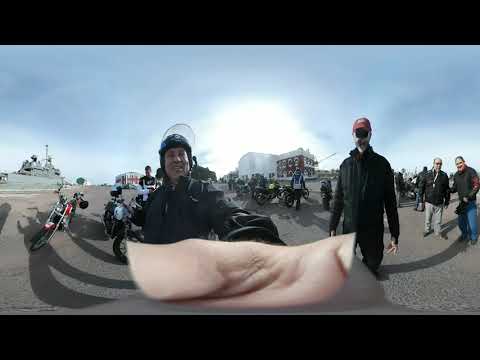The image captures a detailed and somewhat grainy selfie taken by a white man wearing a motorcycle helmet with a flipped-up visor and a black leather jacket. He is standing in front of a group of fellow riders. The man's hand is visible, indicating he pressed the button to take the photo. Surrounding him are several parked motorcycles of varying shapes and models, adding to the scene's dynamic feel. The background reveals a partially overcast sky with hints of blue trying to break through and an intriguing mix of urban and nautical elements. Behind the group, you can see a large naval vessel, likely an old battleship, hinting that they might be at the edge of a pier. There’s also a square red house and other buildings, possibly part of a city or a university campus. Adding to the group dynamic, everyone, primarily white men, is either standing or seated on their motorcycles, smiling, and looking at the camera. The image is framed with black borders at the top and bottom, giving it a vintage or worn feel.